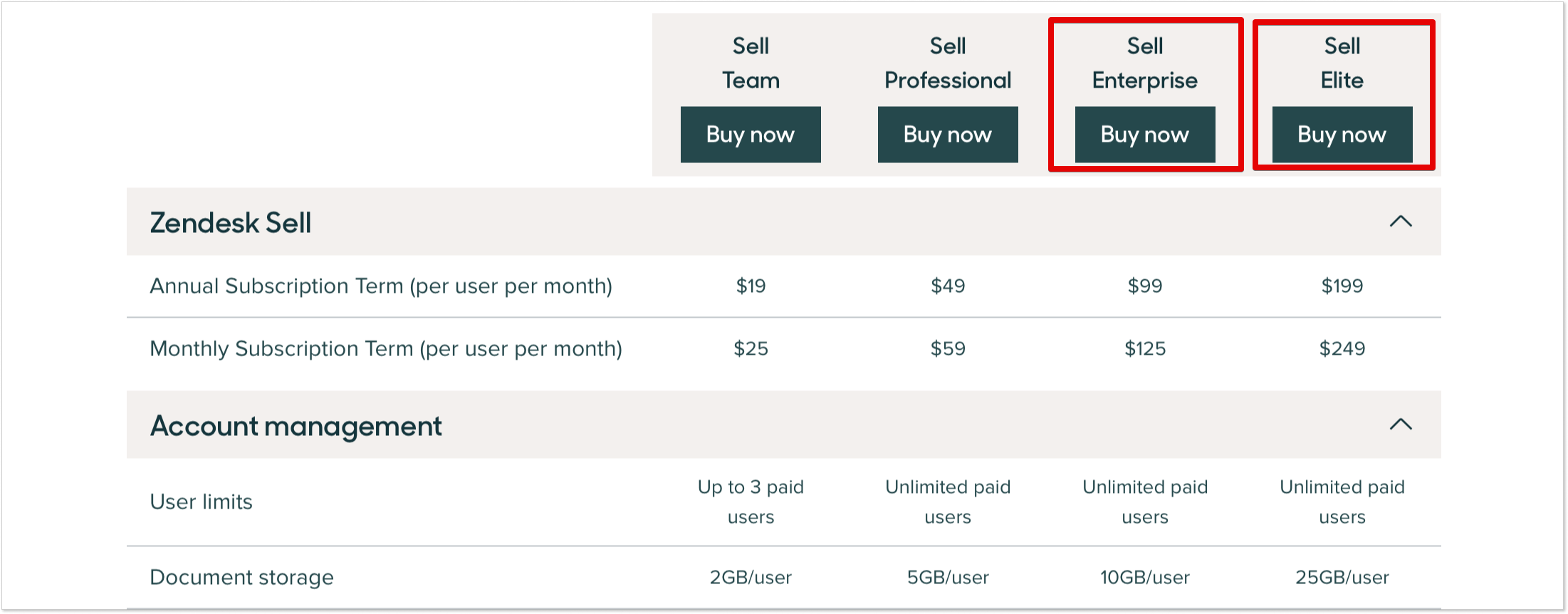Screenshot of a sales website showcasing various subscription plans. At the top right, there are different sections users can select. The categories listed are "Sell Team," "Buy Now," "Sell Professional," "Buy Now," "Sell Enterprise," and "Sell Elite." The last two categories, "Sell Enterprise" and "Sell Elite," are highlighted with a red box. The left side of the image displays a pricing table with text that reads: "Send Desk Sell Annual Subscription Terms per User per Month." The listed prices for the plans are $19, $49, $99, with the two highlighted plans likely having different pricing options.